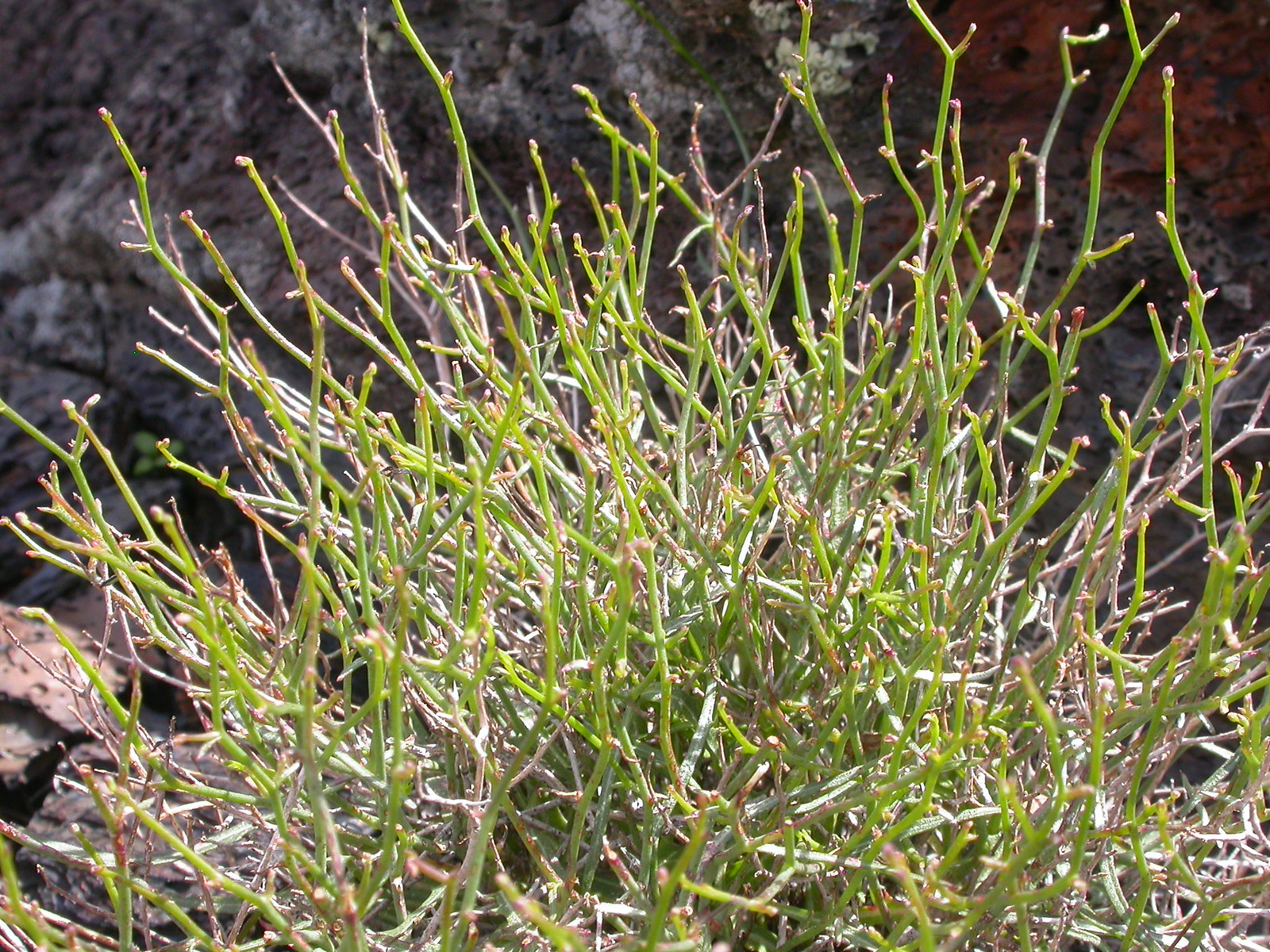This photograph captures a unique, shrub-like plant situated in a rugged, desert-like environment, possibly near low-lying mountains. The plant, central to the image, displays a mix of pink, purple, green, and brown colors with spiky, prickly leaves that suggest it could be painful to touch. Its appearance is somewhat reminiscent of a tumbleweed before it turns completely brown. In the background, a woodsy area leads into a rocky terrain featuring dark and beige stones, along with hints of lighter and possibly red-colored rock, providing a stark contrast to the vibrant plant. The overall scene showcases a blend of natural elements, emphasizing the harsh, yet captivating beauty of the desert landscape.